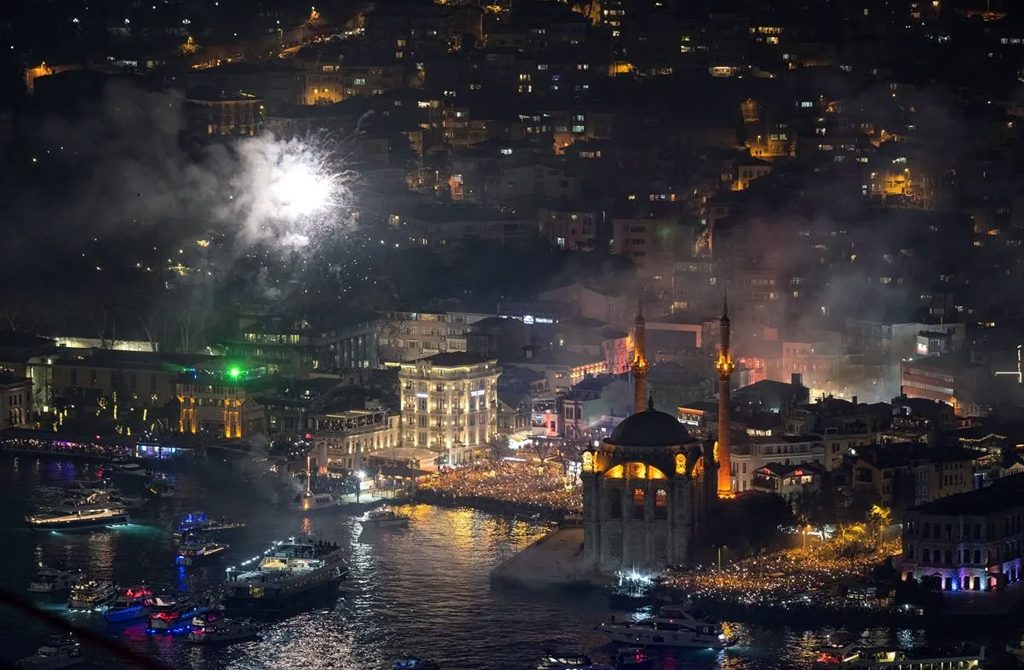The photo captures a vibrant nighttime scene, possibly in Greece, featuring ancient, illuminated waterfront buildings. The city is alive with activity, as a large crowd gathers both on land and on boats in the water, watching a spectacular firework display. Smoke fills the air from the fireworks, with one particularly bright white firework visible on the left side of the frame. The perspective of the shot suggests it was taken from a high vantage point, maybe from a drone or a tall building, capturing the urban center's intricate details. This festival-like atmosphere, reminiscent of international celebratory events, makes the city glow with festive lights amidst the dark night sky.